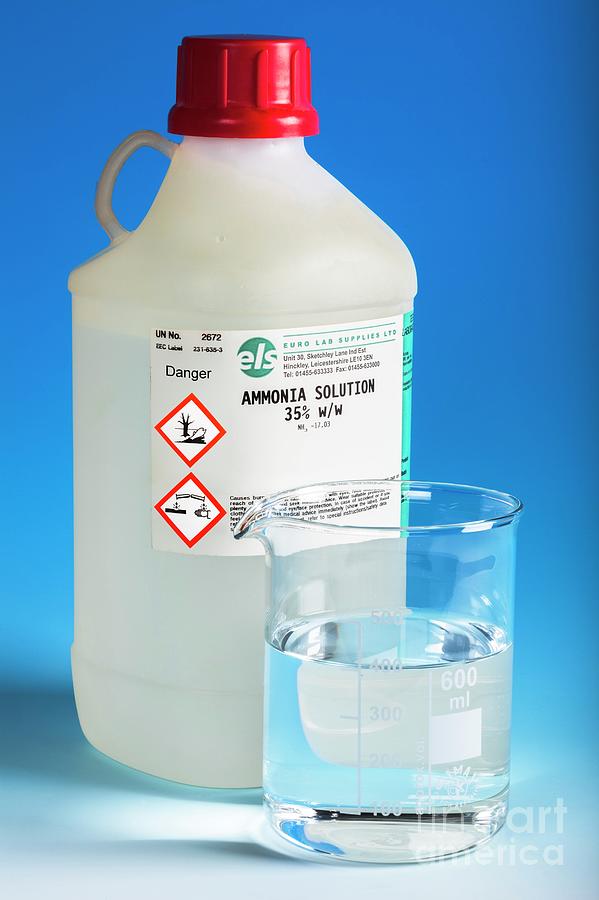Against a gradient blue background that lightens to a bluish-white near the bottom, a large, opaque off-white plastic jug with a bright red cap stands prominently. The front label, which reads "Ammonia Solution 35%," features critical warning symbols, including red diamonds with hazard pictograms and the word "DANGER." The bottle is marked as a product of Euro Lab Supplies. Positioned in front of the jug is a transparent glass measuring cup, filled to the 400 milliliter mark with a clear liquid, likely the ammonia solution. The measuring cup has a spout and white measurement markings. In the lower right corner of the image, the watermark "Fine Art America" is visible.